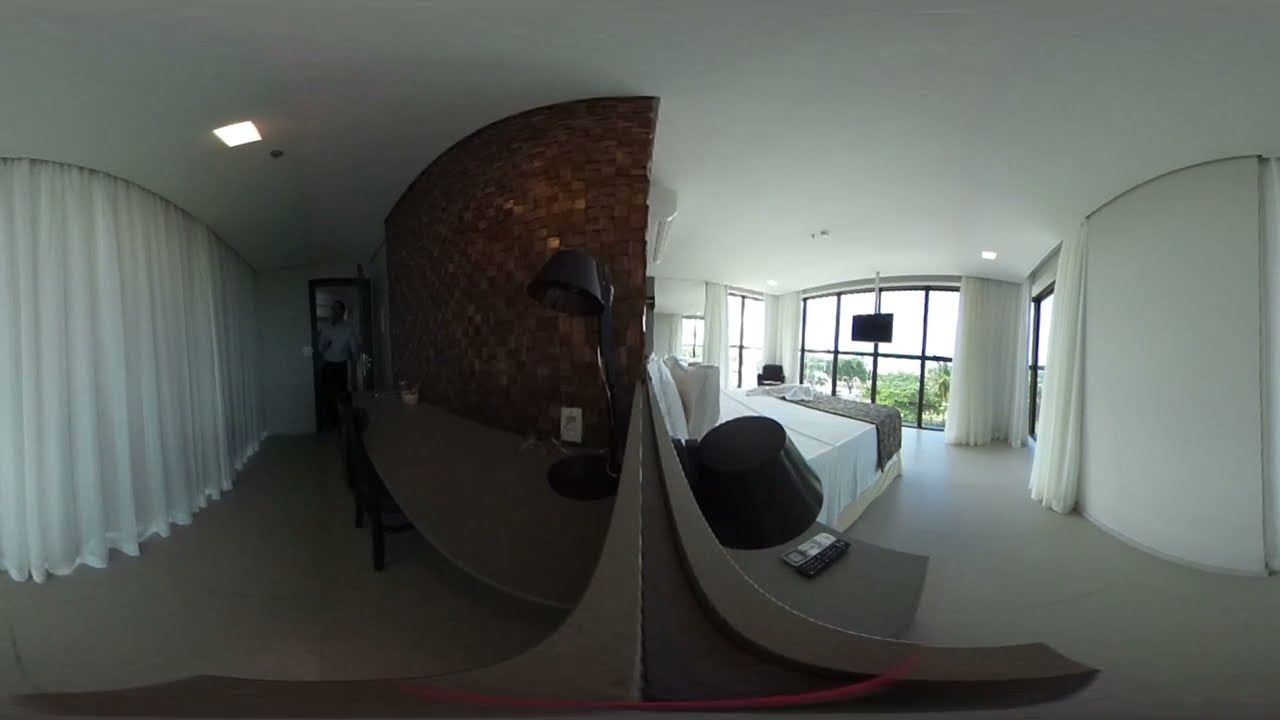The image is a color photograph of a very modern, white house, situated in a tropical environment, and is composed of two photographs pieced together to form a single landscape-oriented shot. The right side of the image features a bedroom with large windows on two sides, one behind the bed and another with floor-to-ceiling white curtains, offering ample natural light. The bed in the room is dressed with white sheets and has a dark bedspread at the end, accompanied by a black rounded tabletop nightstand nearby. Suspended from the ceiling above the bed’s headboard, there is a television mounted in front of the window. On the left side of the image, there is a different room with a brown-checked wall and a countertop, where a man wearing a white shirt and dark pants is seen entering through a door. The ground on the left side is carpeted, contrasting with the harder white flooring on the right. The overall style of the photograph combines photographic representationalism with a panoramic filter, capturing the modern, airy, and sharply defined interior design elements of the space.